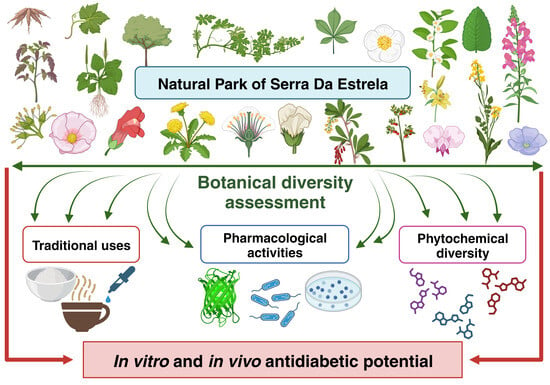The photograph is a horizontally oriented, color illustration that resembles a flyer or a book page. At the center of the image, in a prominent blue box with black letters, it reads "Natural Park of Serra da Estrela." Surrounding this title, colorful, cartoon-like illustrations of a variety of plants and flowers are depicted, including pink and white blossoms, yellow dandelions, cotton-like flowers, ivies, and vines.

Beneath the main illustration, the text "Botanical Diversity Assessment" is displayed. The assessment is divided into three main categories, indicated by bluish-green arrows pointing to various sections within the photo. The first category, "Traditional Uses," shows icons like a coffee cup and a medicine dropper, highlighting the traditional medicinal applications of these plants. The second category, "Pharmacological Activities," is marked by illustrations of pills and Petri dishes, indicative of the medicinal research performed on these plants. The third category, "Phytochemical Diversity," includes a DNA profile, illustrating the unique biochemical compounds found within each plant.

At the bottom of the image, in a pink box with black letters, the text "in vitro and in vivo Antidiabetic Potential" is highlighted, emphasizing the researched antidiabetic properties of the plants featured. The entire illustration provides a detailed and colorful overview of the botanical diversity and the scientific research associated with the Natural Park of Serra da Estrela.